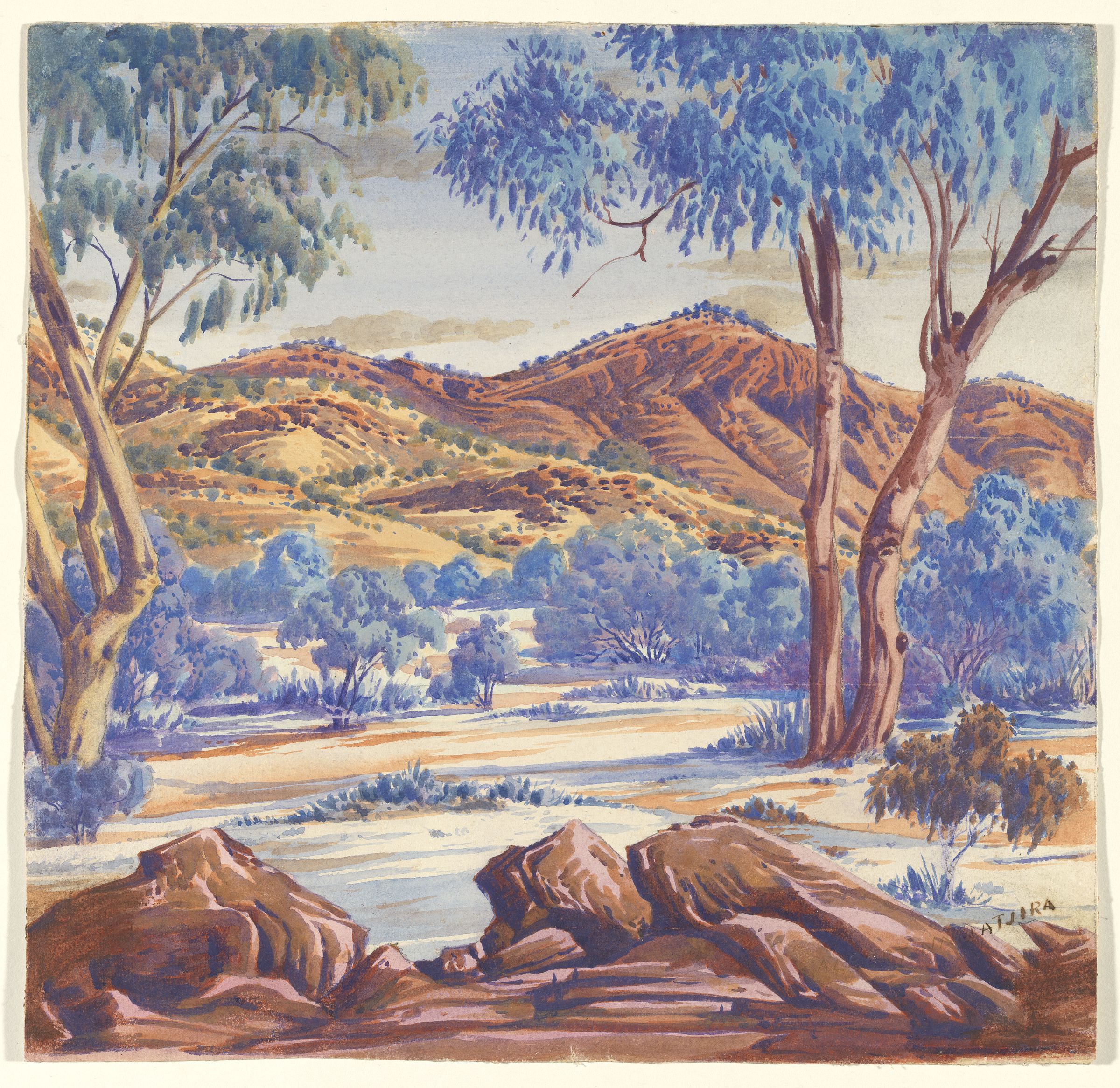The painting is a large square piece bordered by a very light gray or beige, almost like a thin sheet of paper. Depicting a semi-desert landscape, the foreground features rounded brown rocks, some with pinkish tints. Interspersed among the rocks are patches of grass and small green bushes. In the midground, the terrain flattens out with brown soil and shrubs, transitioning into a dense area of blue-tinted trees and bushes. On the far right, there is a crooked tree with a brown trunk and blue leaves, contrasted by a straight tree with green leaves on the left. Tall brown tree trunks flank both sides of the scene. The background showcases light brown hills and darker brown mountains with green shrubs and eroded gullies. Above, a sky with varying shades of light blue and white is dotted by scattered light gray clouds, enhancing the landscape's daytime setting.